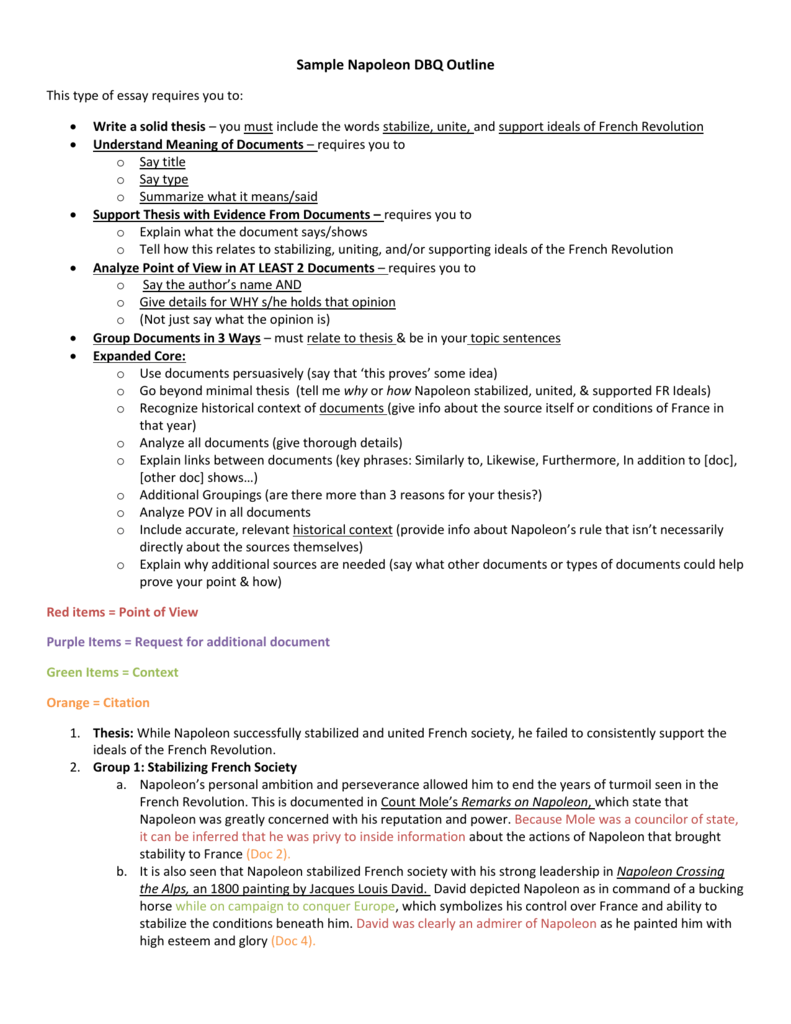This screenshot displays a structured outline for a Document-Based Question (DBQ) essay regarding Napoleon's influence on the French Revolution. The image consists of black text on a white background. At the top, the title "Sample Napoleon DBQ Outline" is emphasized in bold font. Below this, the text elaborates on the essay's requirements, explaining that a robust thesis must include the terms stabilize, unite, and support the ideals of the French Revolution.

The following sections provide detailed instructions for understanding the documents, including identifying the title and type of each document and summarizing its content. The outline underscores the importance of supporting the thesis with evidence from the documents by making clear connections to the concepts of stabilizing, uniting, and supporting revolutionary ideals.

Further, the outline specifies the need to analyze the point of view in at least two documents, recommending the identification of the author's name and a detailed explanation of their perspective rather than just stating their opinion. Additionally, it instructs on grouping documents in three thematic ways that relate to the thesis and should be reflected in the topic sentences.

Towards the end, the "Expanded Core" section suggests using the documents persuasively to demonstrate specific ideas and go beyond a minimal thesis. This section prompts the writer to delve deeper into explaining how and why Napoleon was able to stabilize, unite, and support the principles of the French Revolution.